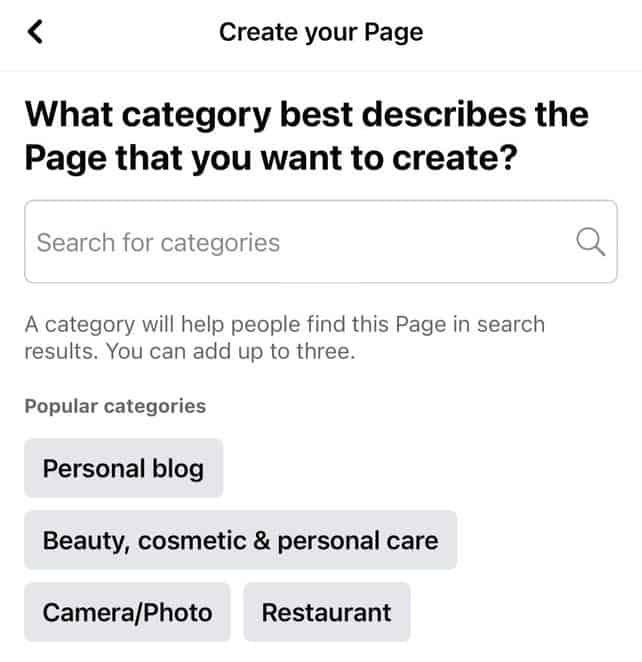The image features a stark, all-white background with a simple, clean layout, primarily in black and varying shades of gray. At the top left corner, there's a black backward-facing arrow, which likely denotes a navigation option. Centered prominently at the top, the black text reads, "Create Your Page." Below this, in the largest font on the page, a question is posed: "What category best describes the page that you want to create?"

Directly beneath the question is a light gray search data field, bordered in gray, with the placeholder text "Search for categories" displayed in gray. To the right of this search field is a small gray magnifying glass icon, symbolizing the search function.

Underneath the search bar, a piece of additional information appears in gray text, stating: "A category will help find this page in search results. You can add up to three." Following this instruction, a section titled "Popular Categories" is listed.

Within this section, four clickable gray buttons are presented, each containing black text with a specific category name:
1. Personal Blog
2. Beauty, Cosmetics, and Personal Care
3. Camera/Photo
4. Restaurant

The entire page is monochrome, featuring only black, white, and various shades of gray. This simple design indicates that the focus is on categorizing pages for probably better search engine optimization (SEO) purposes, although no specific website URL or brand indication is visible.